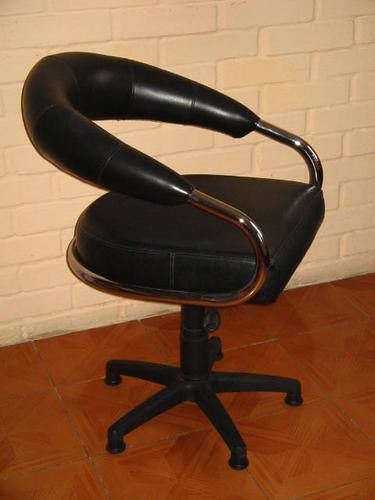The image showcases a black office chair with a unique, wraparound, C-shaped backrest. The chair, which appears to be made of black leather or a similar material, features chrome-colored metal arms that loop around the sides. It has a thick black cushion, approximately four inches tall, for added comfort. The base of the chair comprises five legs equipped with wheels, characteristic of a typical office or desk chair, allowing it to roll easily. The chair is positioned on a brown and orange tiled floor, and it is facing to the right. The background includes an interior white brick wall, providing a stark contrast to the dark chair. The chair also includes a lever beneath the seat for adjusting its height. The setting is simple and devoid of other elements, highlighting the chair's distinct design against the minimalist backdrop.